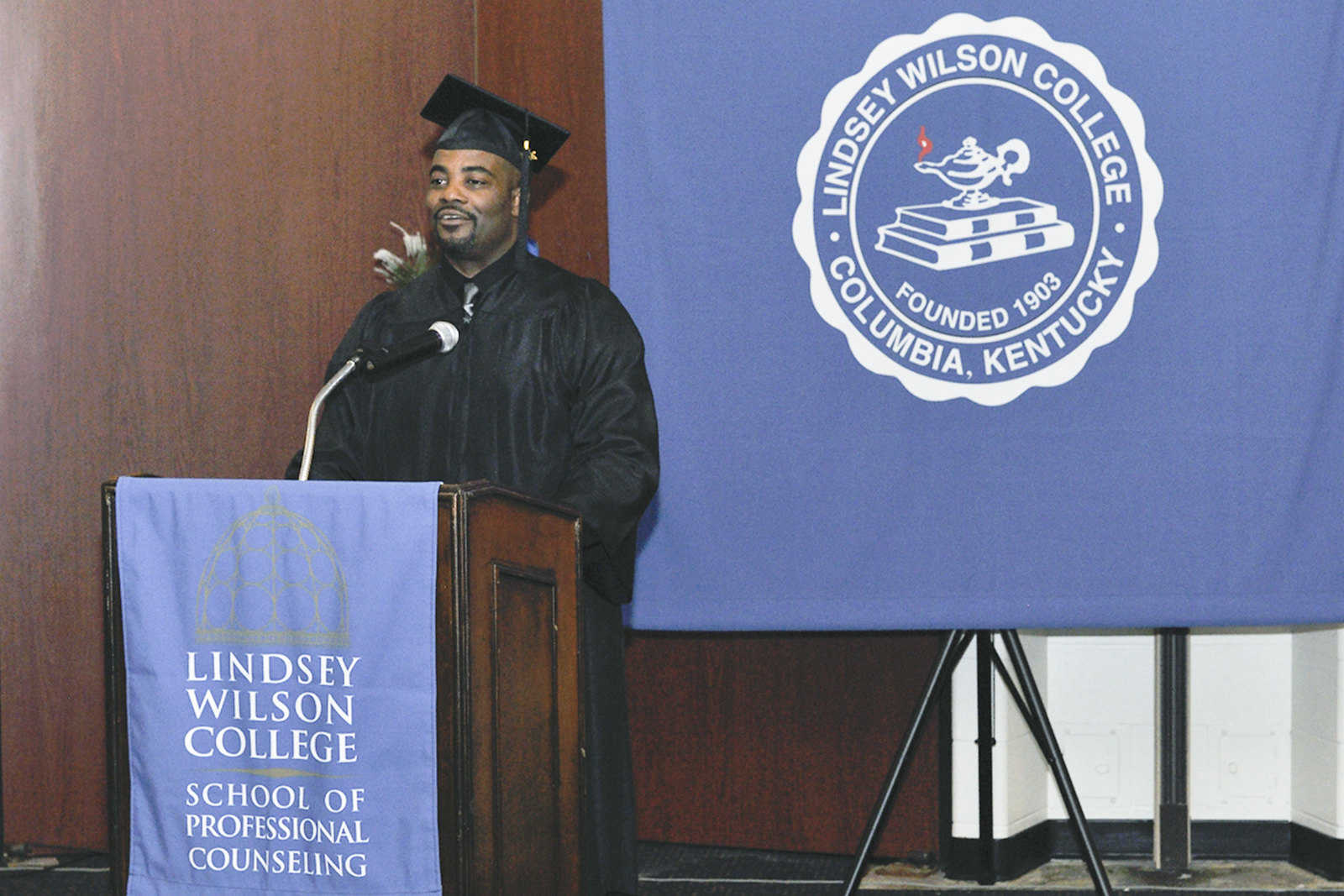In this color photograph, a proud African American man, adorned in a black graduation cap and gown with a silver tie, stands at a wooden podium speaking to an audience. He has a mustache, goatee, and slight stubble, with a visible smile showing a sliver of his teeth. Directly in front of him is a mixed silver and black microphone, and a blue cloth banner on the podium reads, "Lindsay Wilson College School of Professional Counseling." Behind him is a prominent blue banner featuring a white circular emblem that states, "Lindsay Wilson College, Columbia, Kentucky, founded 1903." The emblem features two books topped by a genie lamp with an orange and yellow flame, symbolizing enlightenment and knowledge. An arrangement of blue and white flowers can be seen, adding to the celebratory atmosphere of this significant moment at Lindsay Wilson College in Columbia, Kentucky.